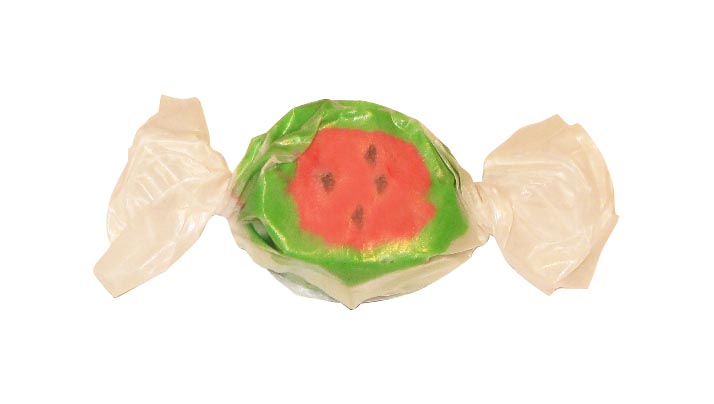In the photograph, there is a piece of saltwater taffy wrapped in matte-finish white wax paper, exhibiting reflections from the light source, indicating a well-lit setting against a white background. The wrapper is twisted tightly at both ends, characteristic of individually wrapped candies. The taffy itself is designed to resemble a watermelon slice, with a bright lime green exterior mimicking the rind, and a vivid pink interior representing the watermelon flesh. There are four small black spots within the pink center, imitating seeds, likely achieved through artificial food coloring. The candy has a circular to slightly oval shape and could be hard or chewy. The taffy creates a familiar rustling noise when unwrapped, enhancing its distinctive charm and appeal.